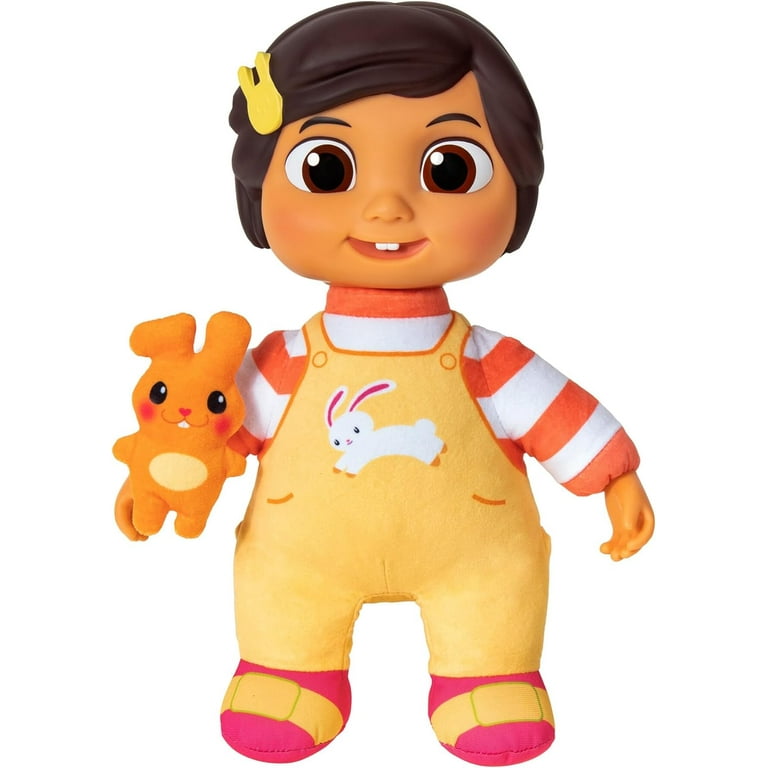This image depicts a life-like doll resembling a young child, ideal for a 4 or 5-year-old. The doll has a round, caramel-colored face with big, expressive brown eyes and a small mouth displaying two front teeth. It features short, dark hair styled with a bang in front, parted on the side, and adorned with a yellow clip. The hair appears to be molded plastic rather than artificial strands. Dressed in an orange and white striped shirt, the doll wears a yellow jumper with orange borders, which has a picture of a white rabbit on the front. The outfit is complemented by pink shoes with yellow straps. In its right hand, the doll holds an orange stuffed rabbit with black eyes, a lighter yellow belly, pink cheeks and nose, and white teeth. This doll, which has arms out to the side, evokes a charming, almost Dora the Explorer-like appearance and suggests a stuffed texture, making it an inviting toy for young children.